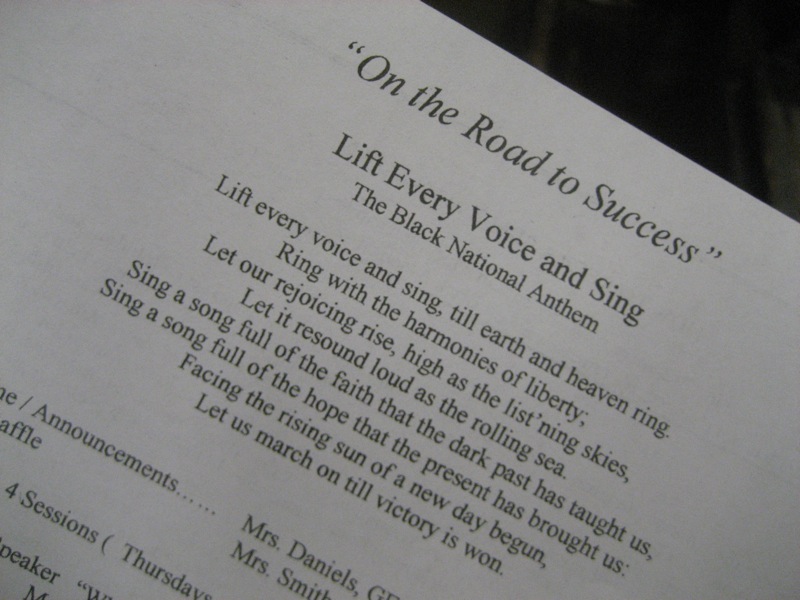The image features a white piece of paper set against a black background. At the top of the paper, in quotation marks, is the title "On the Road to Success." Below the title, the text proclaims "Lift Every Voice and Sing," recognized as the Black National Anthem. The lyrics follow, reading: "Lift every voice and sing till earth and heaven ring. Ring with the harmonies of liberty. Let our rejoicing rise high as the listening skies. Let it resound loud as the rolling sea. Sing a song full of the faith that the dark past has taught us. Sing a song full of the hope that the present has brought us. Facing the rising sun of a new day begun, let us march on till victory is won."

Further down the page, additional text is partially visible, including names like Mrs. Daniels and Mrs. Smith, suggesting a program or announcement format. The document seems to have slanted text, possibly indicating a photograph taken from an angle. Details at the bottom left include a telephone number "47070255." On the top left corner of the paper is a confirmation for a radio reception from Dubai, dated April 14, 1980, with a frequency of 21,485 Hz, and mentions a location in Japan. There's also a blue selector and a stamp, along with the signature of the chief engineer from Dubai Radio and Color Television. The right side of the paper has fragments of text and a blank rectangular box near the top, hinting at what might be a sender or recipient identifier, including names like Nobiyuki Takahashi and Masashino city, Tokyo 180, Japan.